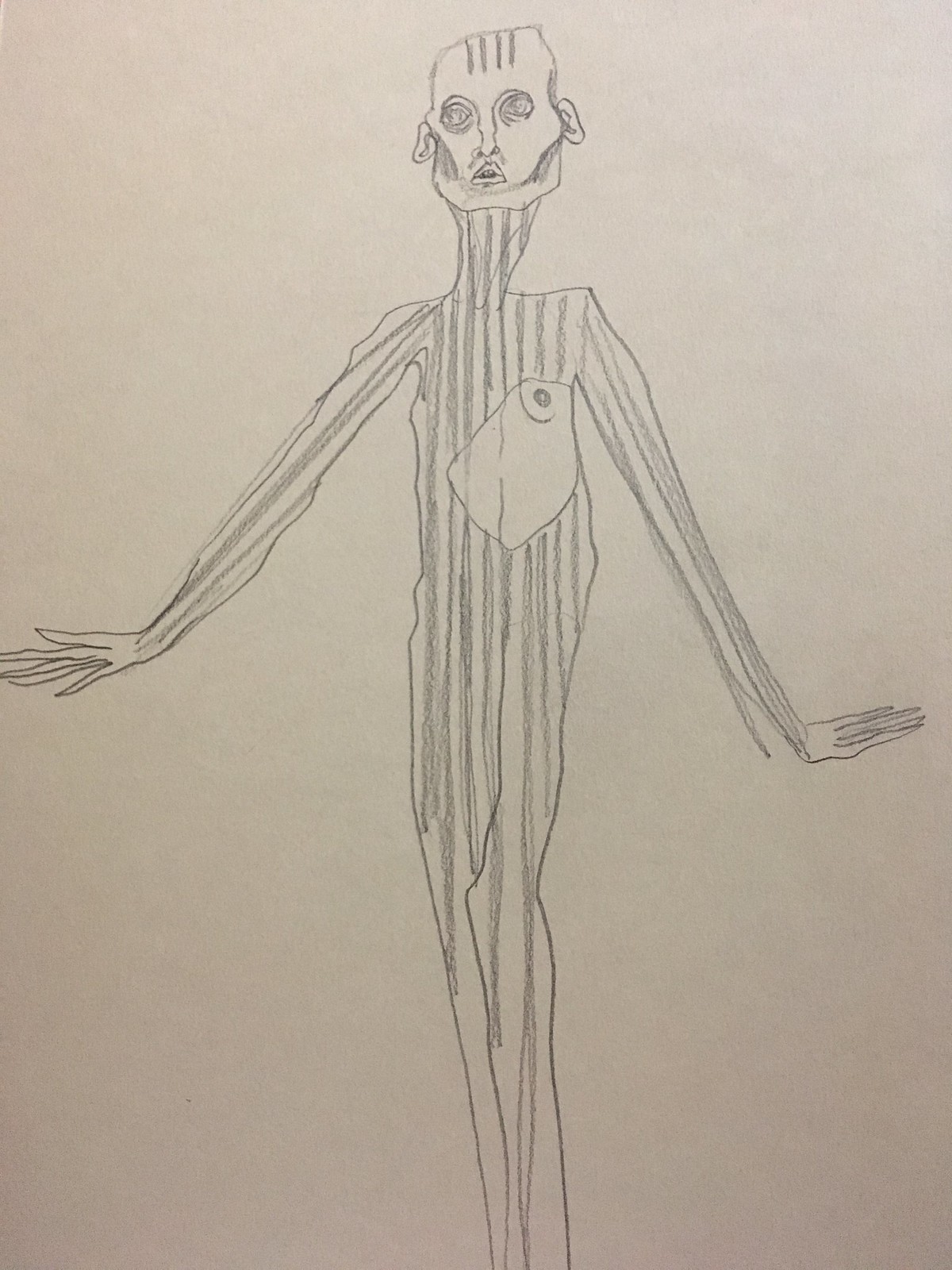This is a pencil sketch of a human-like figure characterized by exaggerated features. The figure has remarkably long arms, legs, and neck, paired with an average-sized, oblong-shaped head. Detailed shading emphasizes its elongated form, with particular attention given to the eyes, which are heavily shaded, and the slightly open, neutral-shaped mouth. The ears are also drawn in at the top of the head, which is accented with four lines suggesting hair or texture. The sketch showcases defined shading along the cheeks and a textured torso. The torso features notable pencil lines against an off-white or gray background, possibly the natural color of the sketch paper. There is a distinct cutout in the center of the torso area that highlights a small, detailed depiction of a human nipple, adding a layer of anatomical precision to the otherwise abstract figure.